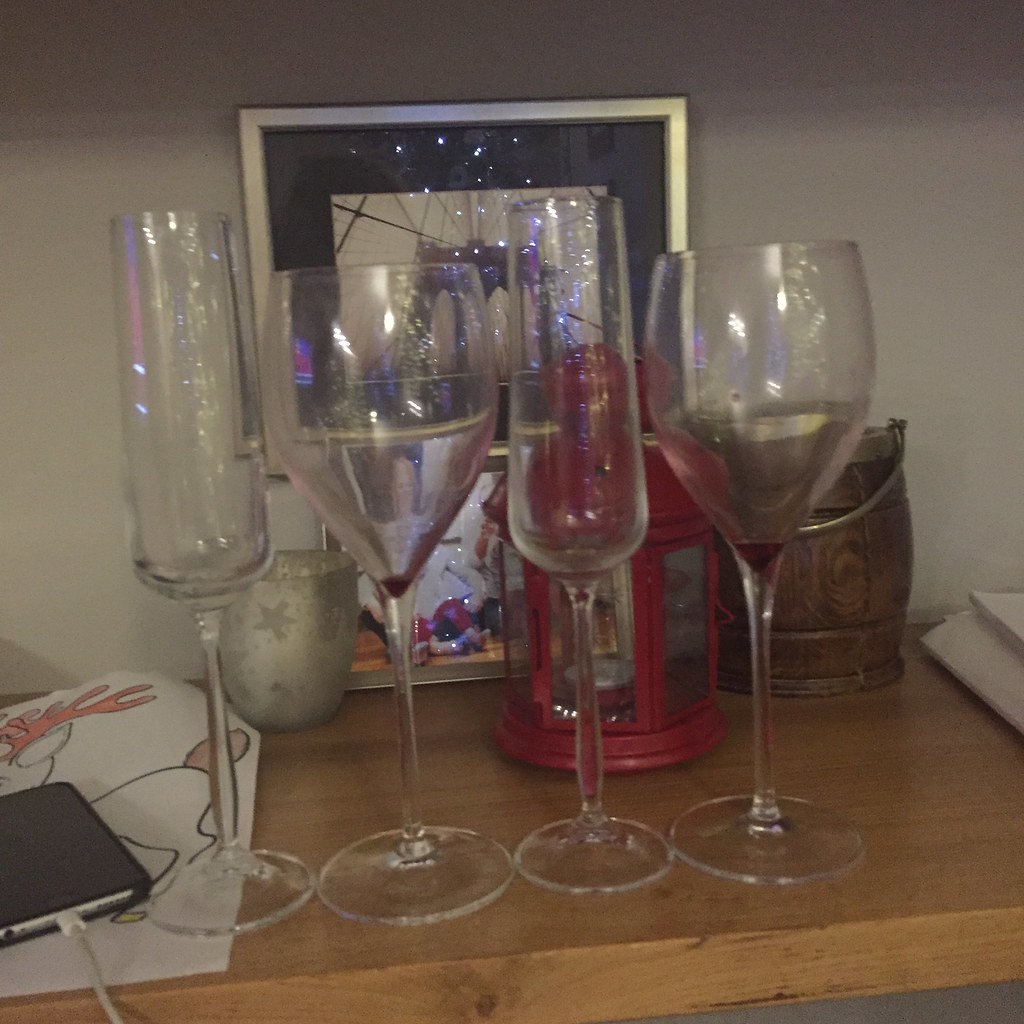This indoor color photograph showcases a neatly organized collection of four wine glasses arranged in a row on a natural wooden shelf. The glasses alternate between two designs: a tall, cylinder-shaped champagne flute and a shorter, wide-bodied wine glass. Behind the glasses, several items are partially visible, including a silver-framed photograph of the Brooklyn Bridge and an assortment of decorative candle holders, one with frosted stars and another resembling a small reddish lantern with glass panels. Additionally, there's an empty bucket-style container with a metal hoop handle and an unfinished coloring book page featuring a partially colored drawing of a deer with antlers. In the lower left corner, a cell phone is being charged, with its white USB cord extending out from the device. The photograph is slightly out of focus and has a dark tone, with a plain white wall serving as the backdrop, adding a minimalist touch to the scene.